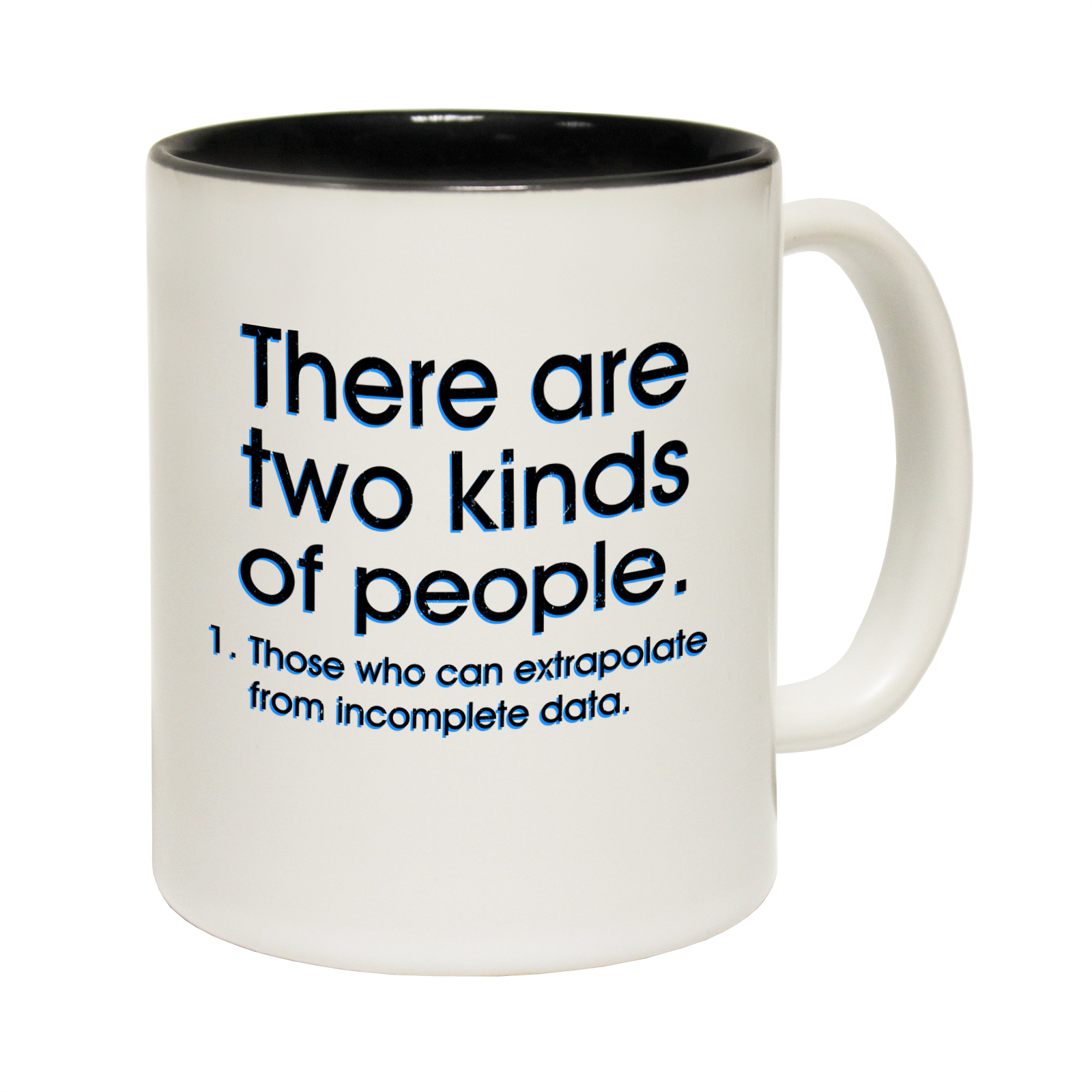This image features a white novelty coffee mug against a solid white background. The mug, viewed from the side, has a black interior and a handle positioned on the right side. The mug's exterior displays a humorous message in bold black text with a subtle bluish undershadow. The text reads, "There are two kinds of people." Below this, in smaller but similarly styled bold text, it continues with "1. Those who can extrapolate from incomplete data," creating a witty implication that the second type of person is understood without being explicitly stated. The mug’s mouthpiece has a slightly reflective surface that catches the light. The simplicity of the mug against the plain white backdrop emphasizes the humorous and clever text design.